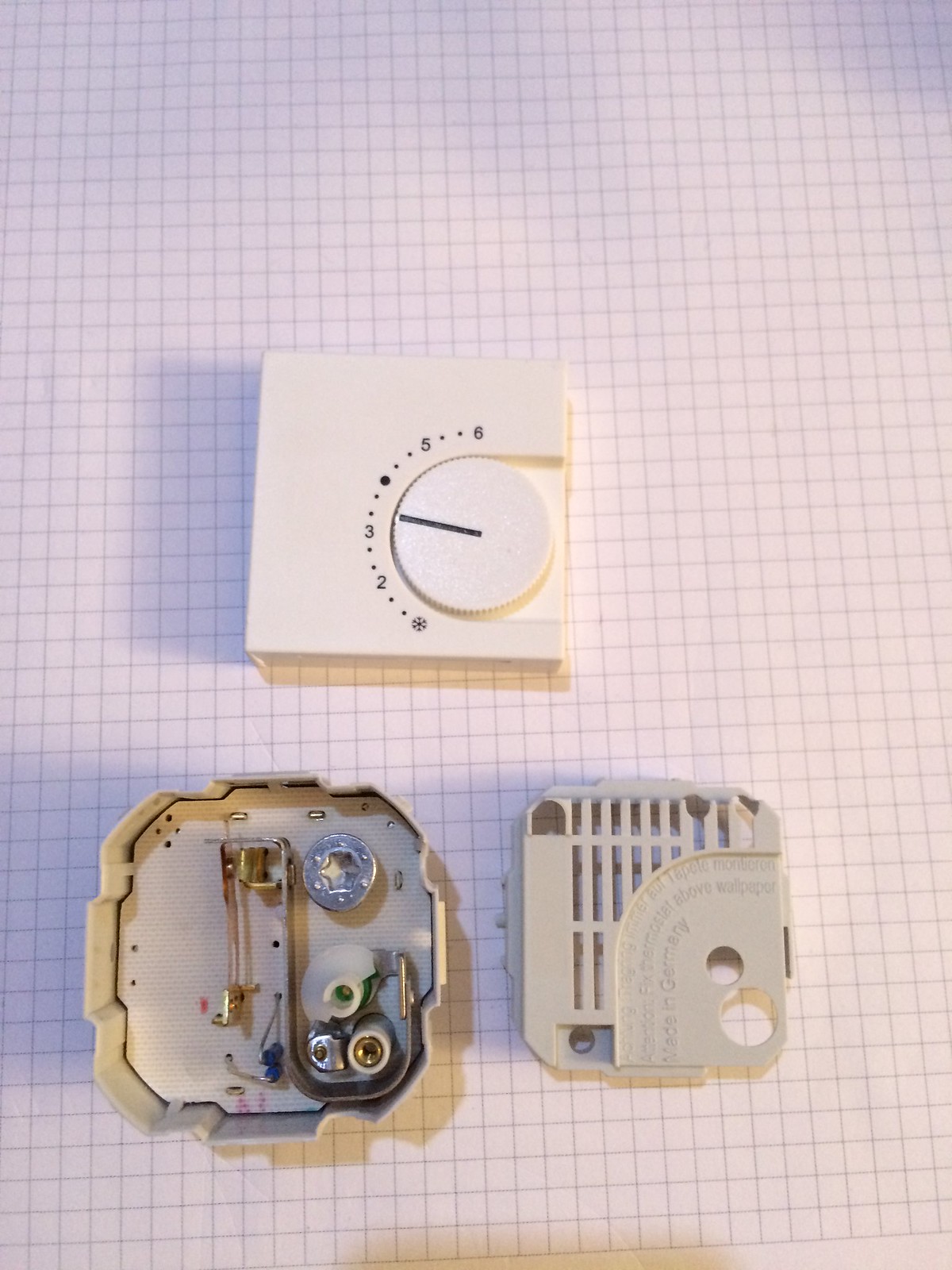The image showcases a disassembled thermostat laid out on a white grid-lined paper background. The grid lines, likely centimeter by centimeter squares, provide a neat and organized backdrop. At the center of the image is the main body of the thermostat, an off-white square box featuring a turn dial on the right side. The dial, marked with a black line to indicate its position, displays various temperature settings ranging from a snowflake symbol to the numbers 2, 3, 5, 6, and a central black dot.

Next to the main body, a smaller square piece with multiple holes for screws is visible, indicating where the thermostat would typically be anchored to the wall. On the left side of the image, the internal components are revealed, including silver and gold-colored metal pieces, a battery-like object, wire connectors, and miniature conduit-type pieces, illustrating the complexity of the thermostat's inner workings.